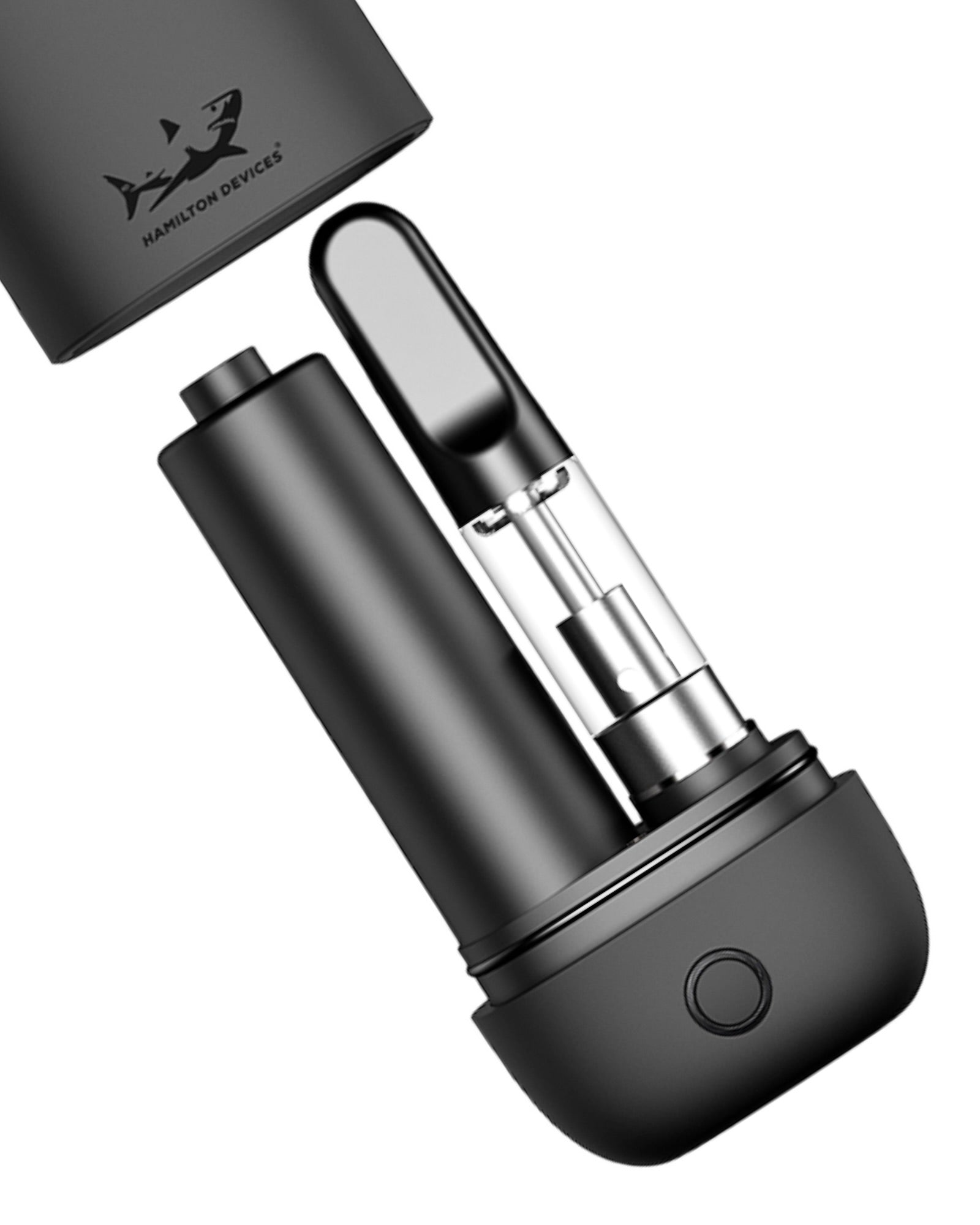This image features a sleek, modern vape device by Hamilton Devices. The vape is predominantly black with stainless steel and silver accents, presenting a sophisticated appearance. The top of the device has a black cap adorned with the Hamilton Devices brand name and a shark logo, which symbolizes the brand's identity. The photograph captures the device at a diagonal angle against a white background, highlighting its compact and portable design.

The vape consists of two main cylindrical sections connected to a base. On the left side is a black metallic cylinder, while the right side features a black cylinder with a flat, tempered top, housing a glass tube section inside. At the bottom of the device, there is a round button, presumably the power button, facilitating easy control of the vape. The overall matte black finish underscores the device's sleek, cutting-edge design, making it a practical and stylish choice for on-the-go use.